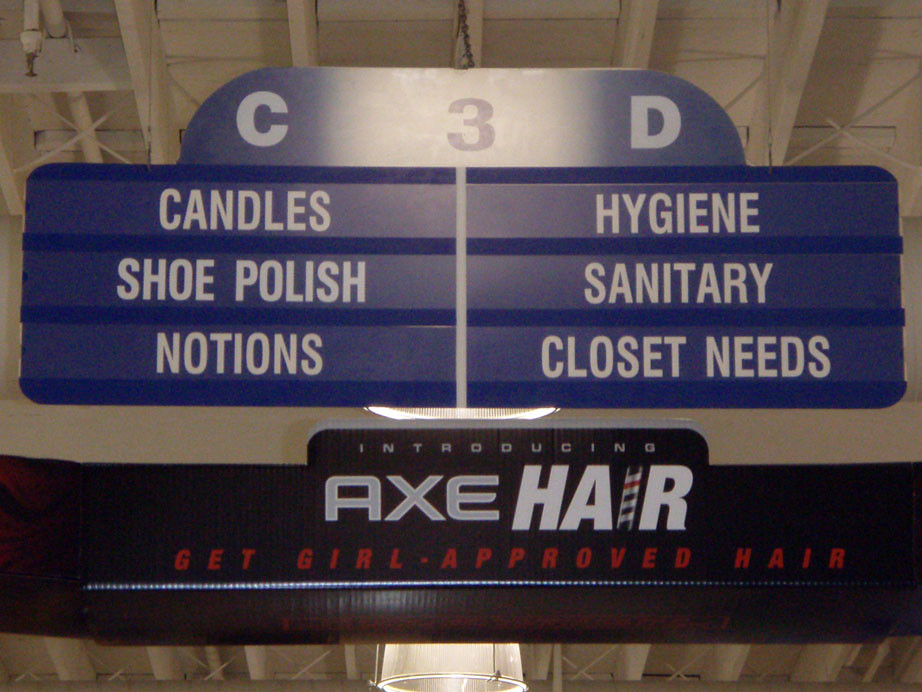The photograph captures a hanging sign in the aisle of a store, prominently featuring a big blue sign at the top with the label "C3D" in white, indicating specific aisle sections. The left side under "C" lists items such as Candles, Shoe Polish, and Notions, while the right side under "D" includes Hygiene, Sanitary, and Closet Needs. Below this blue sign, there's a black temporary sign with white and red print advertising "Introducing Axe Hair," with a barber pole replacing the "i" in "hair," and the tagline "Get Girl Approved Hair" in red letters. The background consists of an open, industrial-style ceiling with visible beams, water pipes, and a sprinkler system, akin to a warehouse environment. A light can also be seen hanging down at the bottom of the frame.